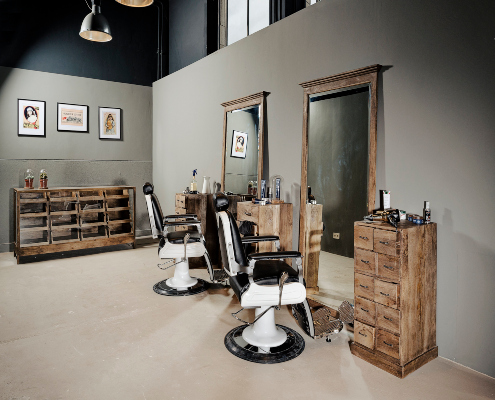The image depicts an old barbershop setup, featuring two black and white barber chairs positioned in front of enormous vintage mirrors, each with a wooden frame. These mirrors, which are as large as doors, reflect the back of the room and contribute to the barbershop's vintage aesthetic. The scene is organized with wooden cabinets flanking the mirrors, adorned with various hair products such as shaving cream and other essentials used for cutting hair. The backdrop includes grayish-pinkish walls, creating an impression of a studio setup with black walls and windows visible above the dividing wall, suggesting an inorganic, staged environment. Additionally, shelves in the background on the left hold framed pictures, contributing to the room's modern and clean decor. Lights from the ceiling illuminate the space, enhancing the overall ambiance.